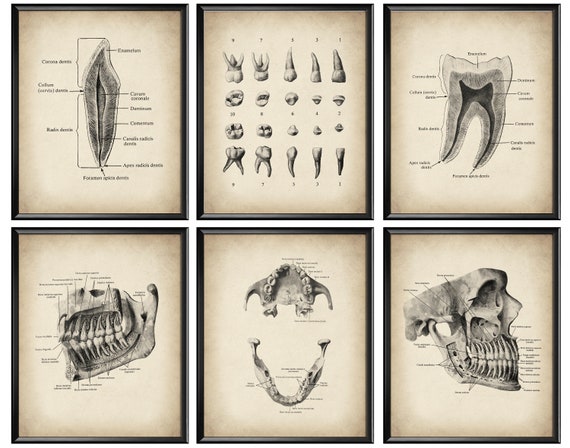The image showcases a set of six highly detailed black-and-white diagrams, presumably extracted from an old textbook. These diagrams primarily focus on various anatomical aspects of the human skull and teeth. Arranged in two rows of three, each drawing is meticulously labeled or numbered, likely for educational purposes. 

- The top left diagram appears more enigmatic, depicting a long midsection of an unidentified anatomical feature.
- The top center illustration displays an array of extracted teeth, each labeled to indicate different types or features.
- The top right diagram offers a detailed cross-section of an individual tooth, with all internal components clearly labeled.
- The bottom left image presents a comprehensive view of the human jaw, illustrating the interaction between the upper and lower teeth.
- The bottom center showcases an overhead perspective of the jawbone and upper teeth.
- The bottom right diagram provides a side view of the entire skull, highlighting how the teeth integrate into both the skull and jaw structure. 

Each diagram is drawn with intricate precision, reflecting a clear intent to educate on dental and skeletal anatomy.